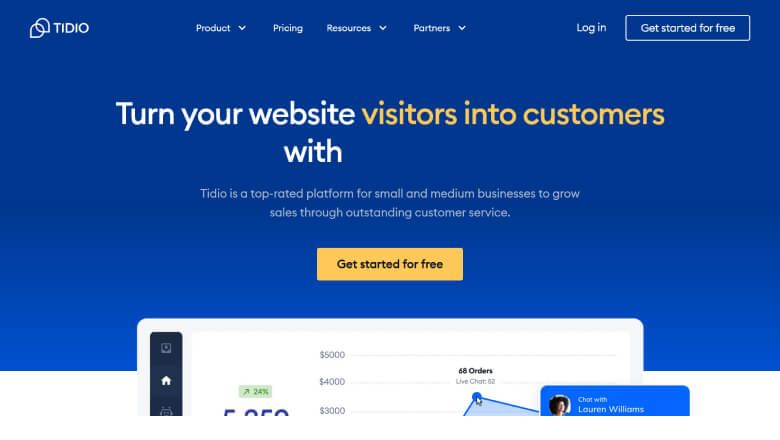The image features a user interface with various sections and elements, including text and graphics. 

In the top left corner, a list includes "TDO", "End Product", "Pricing", "Resources", and "Partners". Below this list are buttons for "Log In" and "Get Started for Free". 

A prominent bar beneath these elements reads, "Turn your website visitors into customers." Accompanying this text is a yellow highlight specifically saying, "Visitors into customers with."

Further description includes a statement that "TDO was the top-rated platform for small and medium businesses to grow sales through outstanding customer service." This proclamation is underscored by another yellow rectangle emphasizing "Get started for free."

The lower part of the interface seems to depict a tablet or iPad displaying analytical data and statistics. To the left of this section, there is a column indicating percentages with figures such as "24%". Below this, financial amounts are listed: "$5,000", "$4,000", and "$3,000", along with the note "60 orders" and "live chat." 

A cursor points towards a specific spot on the screen, all set against a predominantly white background. 

Overall, the image showcases various tools and options available through the TDO platform, emphasizing its benefits for enhancing customer engagement and sales.